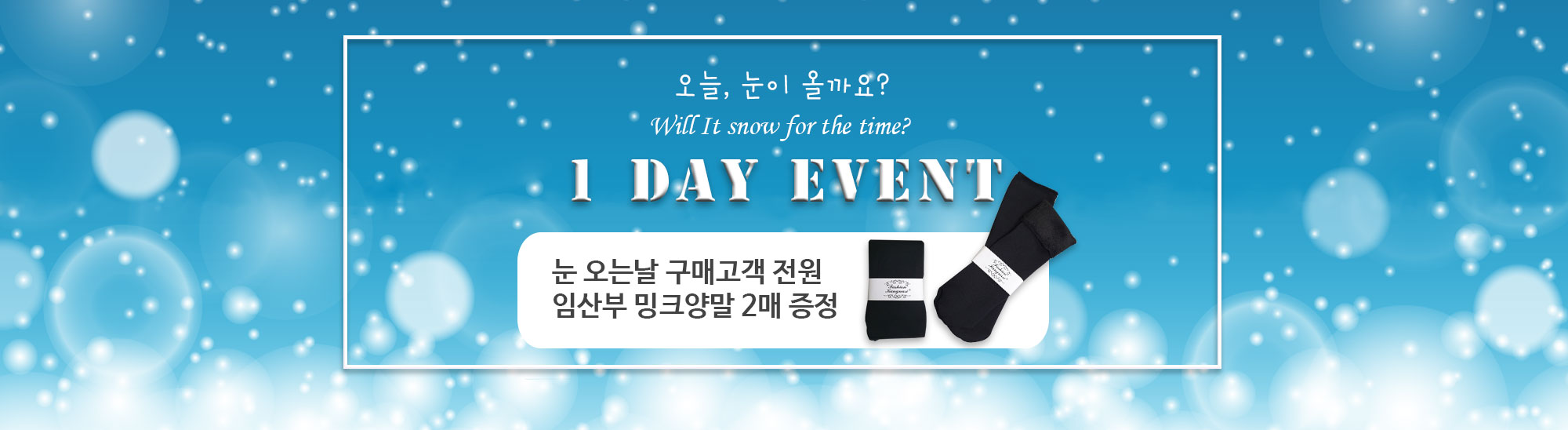The advertisement, primarily written in Korean, showcases a "One-Day Event" with prominent white text centered on the image. Above this text, in smaller font, it asks, "Will it snow for the time?" The Korean text for this phrase is also displayed just above. Situated below the main event text is another line of Korean characters. To the right, two pairs of black socks are showcased—one laying flat and the other slightly angled—each with a white band around the center. The entire advertisement is framed with a white border, creating a boxed-in effect. The background features a blue sky adorned with glowing, translucent bubbles and larger white orbs, evoking a snowy, winter-like atmosphere, enhancing the abstract winter theme of the event.